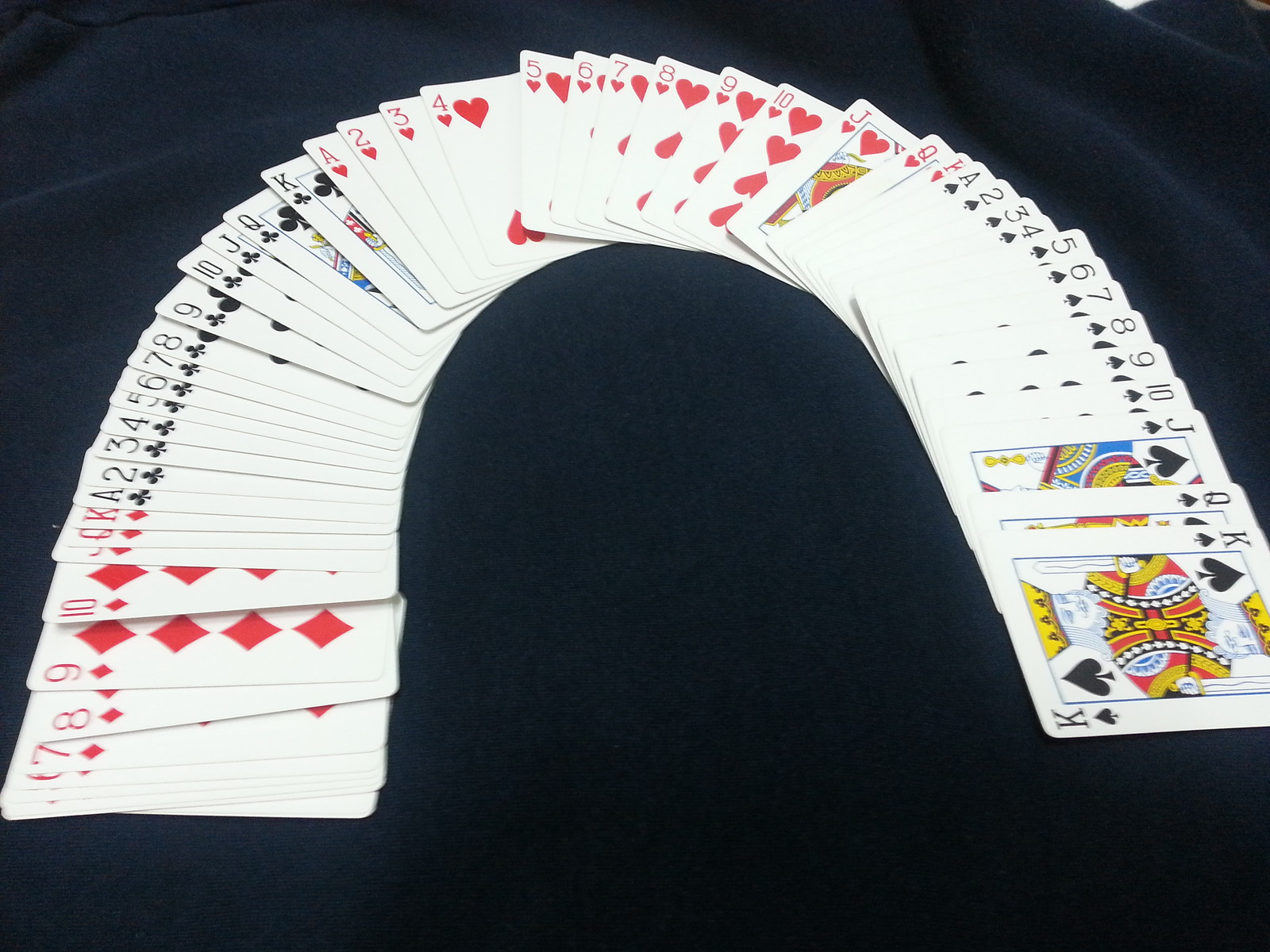A meticulously arranged deck of cards is spread out in a clockwise formation on a large blue surface. The cards begin at the bottom left corner, curving upwards around the top and descending down the right side. The fabric beneath the cards has slight wrinkles just outside the spread.

Starting initially with an Ace of Diamonds hidden beneath other cards, the first visible card is the Seven of Diamonds. As the spread continues clockwise, the sequence includes the Diamonds followed by the Ace of Clubs. The Clubs are displayed clearly from the Ace to the King.

Moving further, the Ace of Hearts emerges next, displayed up to the Queen, with the King slightly peeking out as the spread curves over the top moving to the right side. Following this, the sequence showcases the Ace through King of Spades. Only the edges of the Ace through the Five of Spades are visible in the bottom left corner, slightly overlapped by other cards, followed by a partial view of the Six. The Jack of Diamonds is slightly obscured behind the Queen.

The Clubs are evenly spaced, while the Hearts exhibit larger gaps between the Four and Five, and between the Ten and Jack, creating noticeable spacings. The King of Hearts is partially hidden under the Ace of Spades. Finally, the Spades display closely placed cards except for a small gap between the Jack and Queen.

Overall, the arrangement creates a visually engaging display of the deck, with varying degrees of spacing enhancing the spread's dynamic appearance.